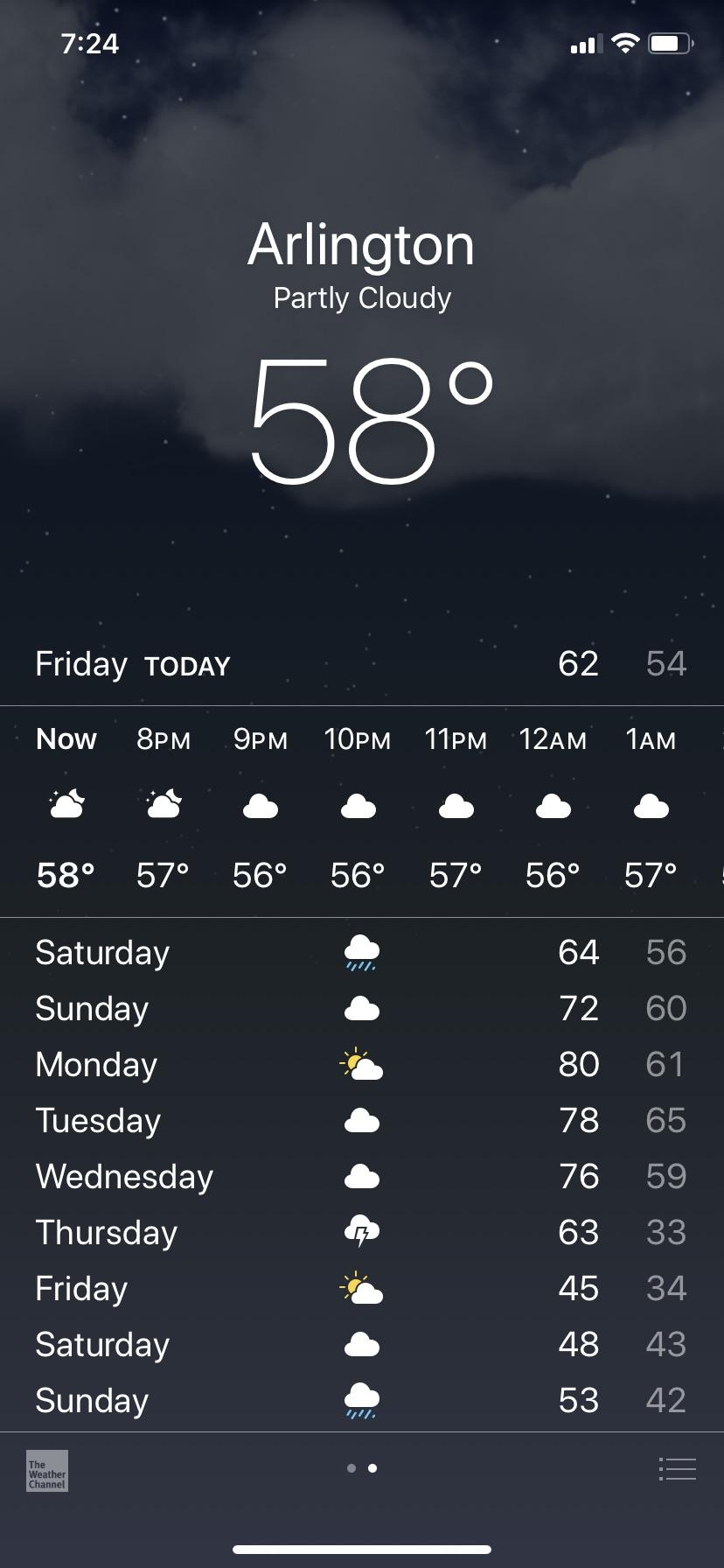A screenshot of a smartphone weather app interface displaying detailed weather information. The background is predominantly black with subtle cloud imagery towards the top. At the upper left corner, there are status icons showing the time (7:24 AM), while the upper right corner displays WiFi and battery status icons.

Centrally positioned, the weather summary indicates the location as Arlington with a current condition of partly cloudy and a temperature of 58°F. Today is Friday, with forecasted high and low temperatures of 62°F and 54°F, respectively.

Below this summary, there is a time series from 8 PM to 1 AM, each hour marked with cloud icons and corresponding temperatures gradually ranging from 58°F to 57°F. Further down, an extended forecast is provided, listing daily predictions from Saturday through the next Sunday. Each day is accompanied by icons representing sun and cloud conditions, as well as high and low temperatures. For example, Saturday shows a high of 64°F and a low of 56°F, while Sunday forecasts a high of 72°F and a low of 60°F.

At the bottom of the screen, there is a small square icon, likely the logo of the weather channel, though it is not entirely legible. The lower left corner features two dots, possibly indicating a pagination element. On the right side of the bottom section, a hamburger menu is faintly visible. A horizontal bar extends across approximately one-third of the screen width at the bottom, suggesting a navigation or status bar.